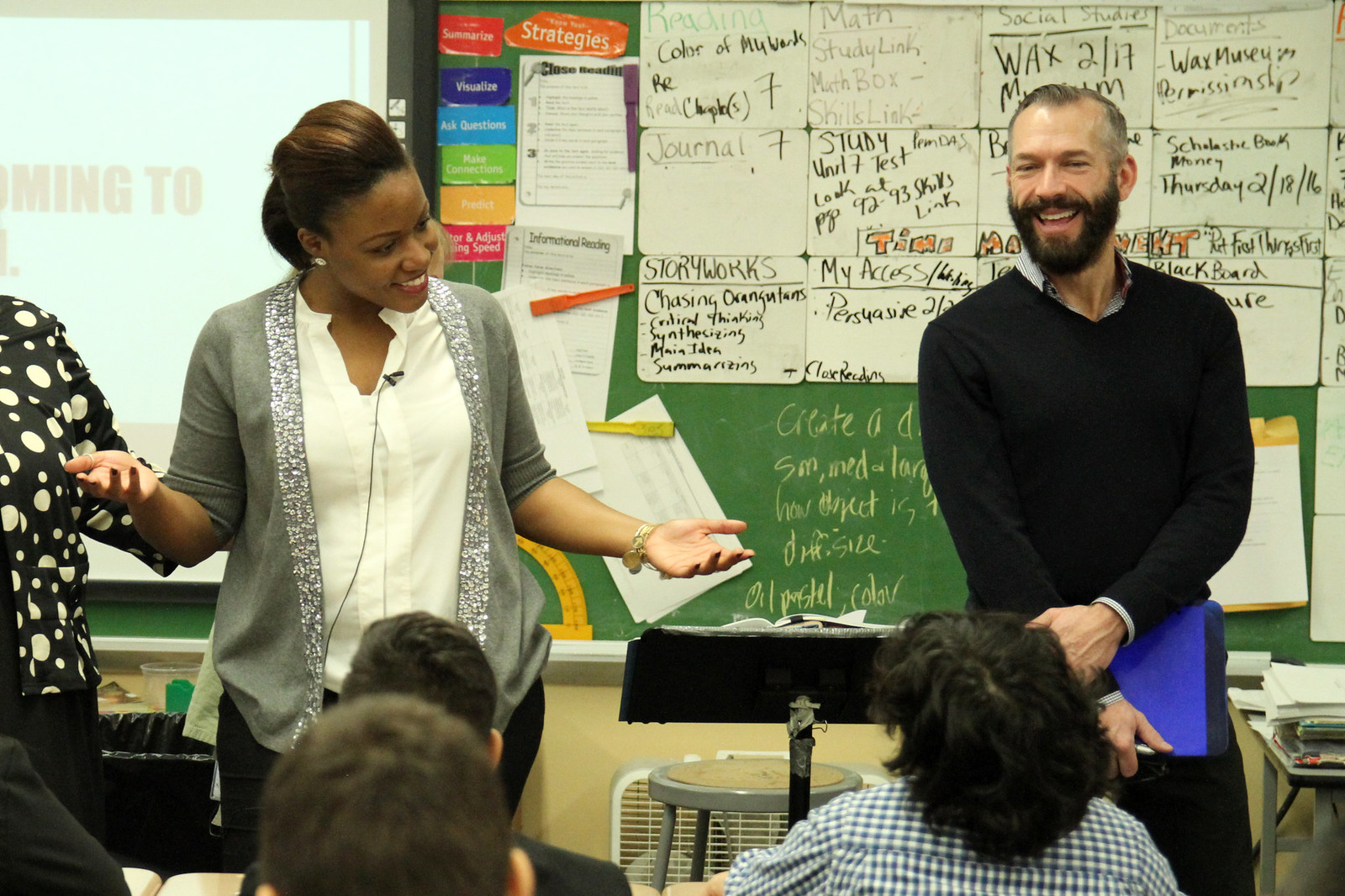In this photograph, a classroom scene is depicted where three individuals are standing at the front. On the far left, partially out of the frame, there is a woman wearing a black blouse adorned with white dots; only her shoulder and chest are visible. Next to her, towards the center, stands a black woman dressed in a white button-down shirt layered with a gray sweater. To her right is a white man with dark hair and a thick beard, clad in a blue collared shirt topped with a black sweater and dark pants.

The backdrop of the scene features a chalkboard filled with extensive writing, as well as various papers and colored printouts taped prominently across its surface. In front of the trio, a group of students is seated at their desks, attentively engaged in the activity led by the presenters.

A black podium, situated between the man and the woman in the center, supports a collection of papers and books. Just behind this podium, a silver stool is visible, accompanied by a white mechanical fan stationed further back. To the right of the man, a desk can be seen, piled high with stacks of paper, contributing to the organized yet bustling atmosphere of the classroom.